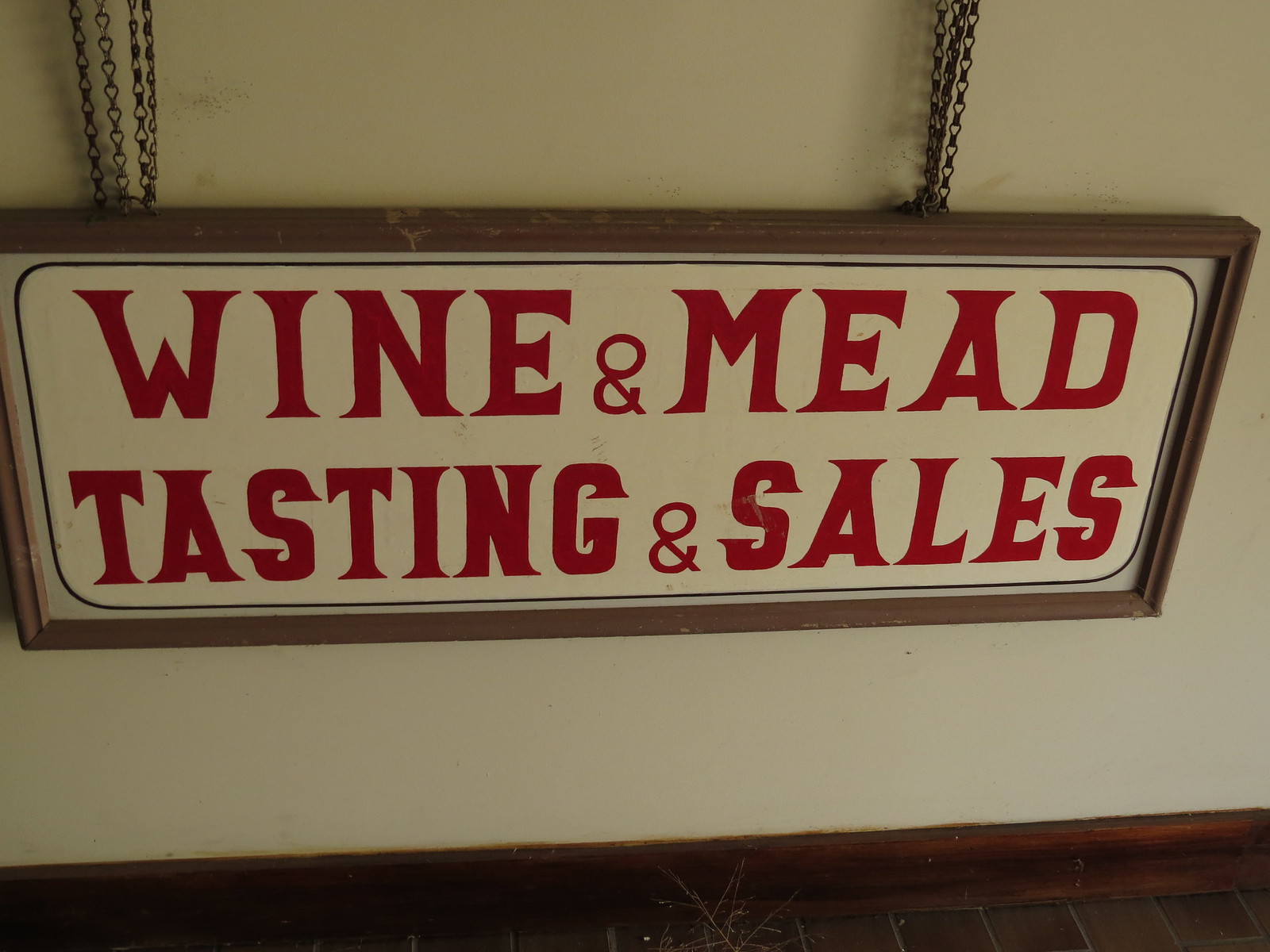The image showcases a horizontally oriented wooden sign with a white rectangular base and an oval-shaped text area displaying "WINE & MEAD TASTING & SALES" in dark red, capital letters. The sign is framed with a wooden border and is suspended from the ceiling by four metal chains on each side. The background features a plain white wall with dark stained wooden crown molding along the bottom. Additionally, a wooden or wood-like tiled floor is visible in the lower part of the image. The overall setting is simple and rustic, highlighting the sign as the focal point.